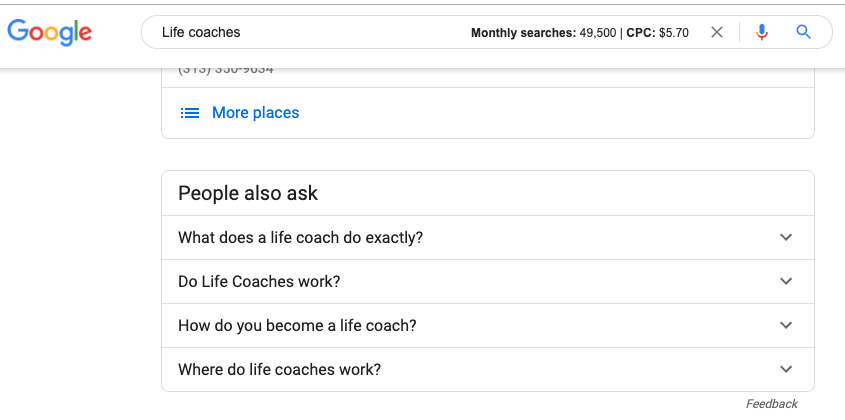The image depicts a Google search results page predominantly featuring a clean, white background. The font across the screen is primarily black, with certain elements, such as a link, displayed in blue, and the iconic Google logo in its vibrant signature colors of blue, red, yellow, blue, green, and red. 

At the very top, there is a navigation bar bordered by dark gray lines. The left side of the navigation bar prominently displays the Google logo. Below this bar is the search query box; it contains the text "Life Coaches" on the left side, while on the right side, statistics about the query are presented: "monthly searches 49,500 CPC $5.70." Accompanying the search bar are the recognizable icons: an 'X' for clearing the search, a microphone symbol for voice search, and a magnifying glass icon for executing the search.

Directly beneath the search bar, the beginning of the search results can be observed. The screen shows a partially visible result that has been scrolled up, rendering its text unreadable. However, below this blur, there is a horizontal triple-line menu icon alongside a clickable option labeled "More places" in blue.

Following this clickable option, there is some white space, leading to a light gray-outlined block marked "People also ask." This section lists related questions, each accompanied by a drop-down arrow to the far right. These questions include: "What does a Life Coach do exactly?", "Do Life Coaches work with", "How do you become a Life Coach", and "Where do Life Coaches work." At the lower edge of this block, the word "Feedback" is displayed in italics on the far right side.